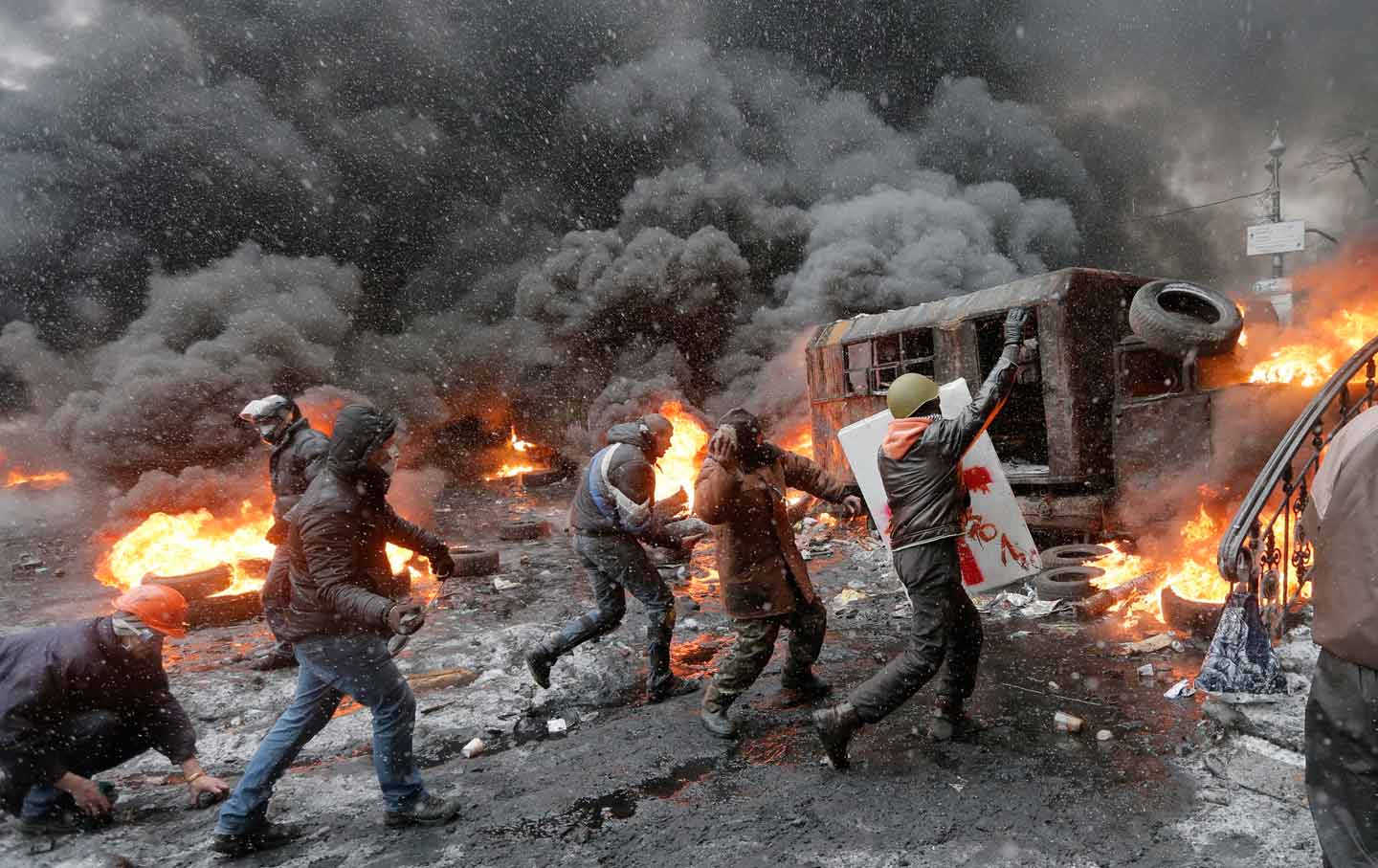The photo depicts a chaotic and intense outdoor scene, likely taken during a riot or a conflict. There are about half a dozen people, some dressed in winter coats, hoods, and helmets, amidst a landscape marred by destruction. Fires blaze throughout the area, producing thick, black smoke that fills the air. The ground is charred, wet, and speckled with ash and rubble, including burned-out vehicles and discarded tires. One person on the right holds a white board as a makeshift shield, while another with a hard hat appears to be in the act of picking up a rock, possibly to throw it. A large truck covered with a tarp blocks the way, contributing to the sense of obstruction and turmoil. A prominent staircase stands incongruously among the devastation, hinting at the remnants of a formerly intact structure. The image vividly captures the aftermath of a significant and destructive event, whether it be an outbreak of civil unrest or a scene resembling warfare.